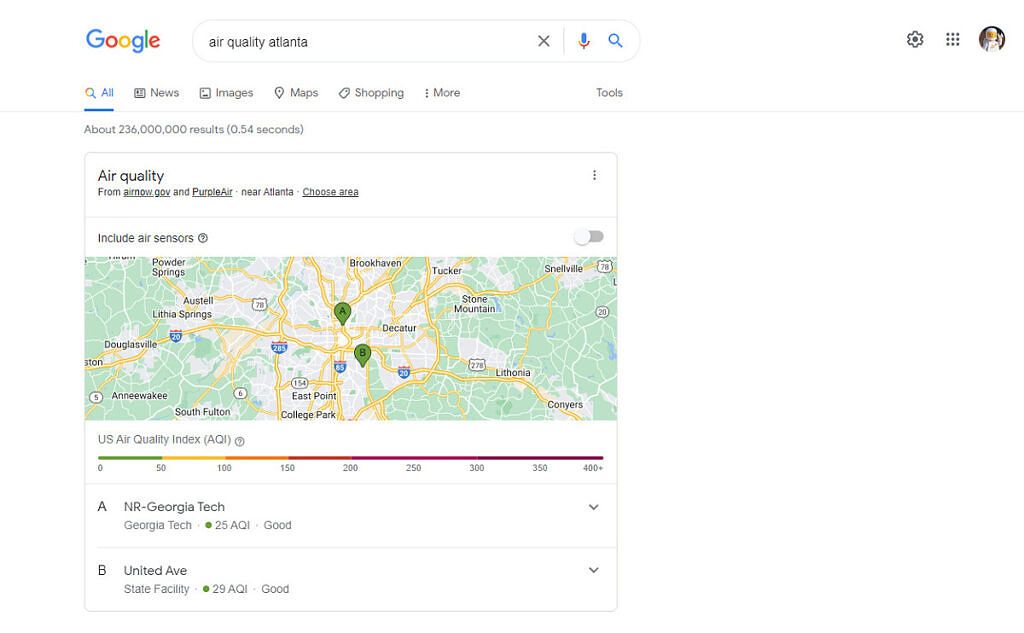Screenshot of a Google search for "Air Quality Atlanta". The Google logo, featuring its recognizable multicolored letters, is positioned on the left followed by a white, rounded search box outlined by a gray border. Inside the search box, in black letters, is the query "Air Quality Atlanta". Accompanying the search box are an 'X' icon for clearing the input, a colored microphone symbol for voice search, and a blue magnifying glass icon for initiating the search.

Below the search box, the standard Google search tabs are visible: All, News, Images, Maps, Shopping, More, and Tools on the far right. The results counter indicates approximately 236 million results returned in 0.54 seconds. The search results prominently feature air quality data sourced from airnow.gov and Purple Air for areas near Atlanta, along with an option to "Choose Area" and an inclusion setting for "Air Sensors".

Beneath, there's a detailed map of Atlanta, showcasing standard mapping colors: yellow for interstates, green for counties, and white or gray for cities. Two green location icons marked "A" and "B" pinpoint specific air quality monitoring sites: "A" located near Georgia Tech and "B" on United Avenue, both providing data according to the Air Quality Index.

In the upper-right corner of the page are three icons: a settings icon, a grid of nine dots (arranged in three rows and three columns), and the user’s personal icon, represented by a circular image resembling a Lego figure in a white suit.